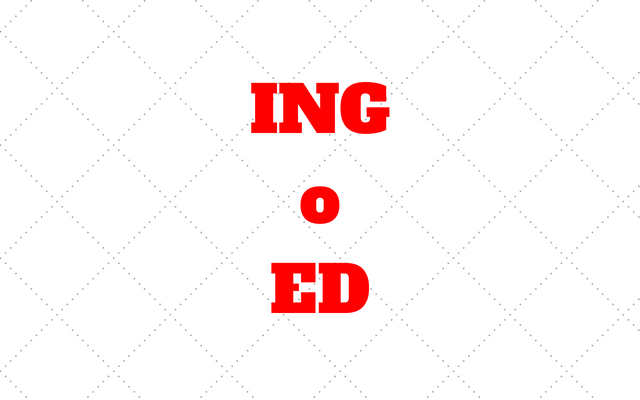The image features a stark white background adorned with a faint, perforated diamond pattern formed by diagonal dotted lines running from the top left to the bottom right corner. This subtle pattern creates a grid of diamond shapes. Centrally positioned on the background are three lines of bold, capitalized red text. The first line displays the letters "ING," the middle line, slightly smaller than the others, simply shows "O," and the third line reads "ED." The overall composition is minimalist and focuses on the striking contrast between the white, patterned background and the vivid red text.